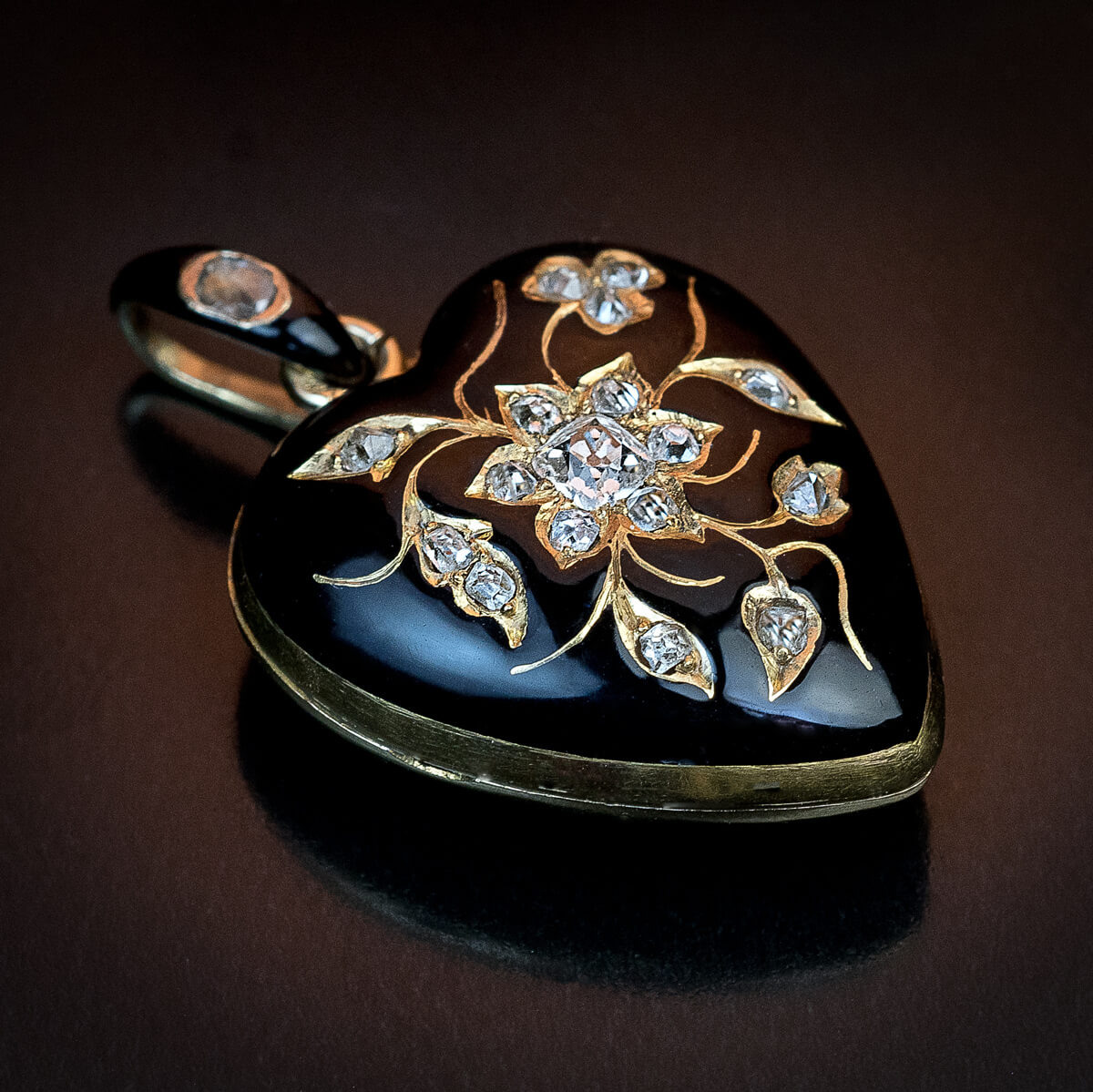The image showcases a heart-shaped pendant, dark brown to black in color and exhibiting a glossy, shiny finish. The pendant is adorned with a gold trim along its border, giving it a luxurious touch. At the top, there's a prong or metal hoop that features a small diamond, which is likely the attachment point for a chain, emphasized by a subtle gold ring.

The pendant's face is intricately engraved with a floral design, featuring a flower-shaped central diamond encased in gold lining. The flower is elegantly surrounded by stem-like, curling extensions that form leaf patterns, each inlaid with tiny diamonds, adding to the pendant's intricate and sparkling detail. The backside of the pendant reflects its glossy nature against a plain brown background, adding depth to the overall image.